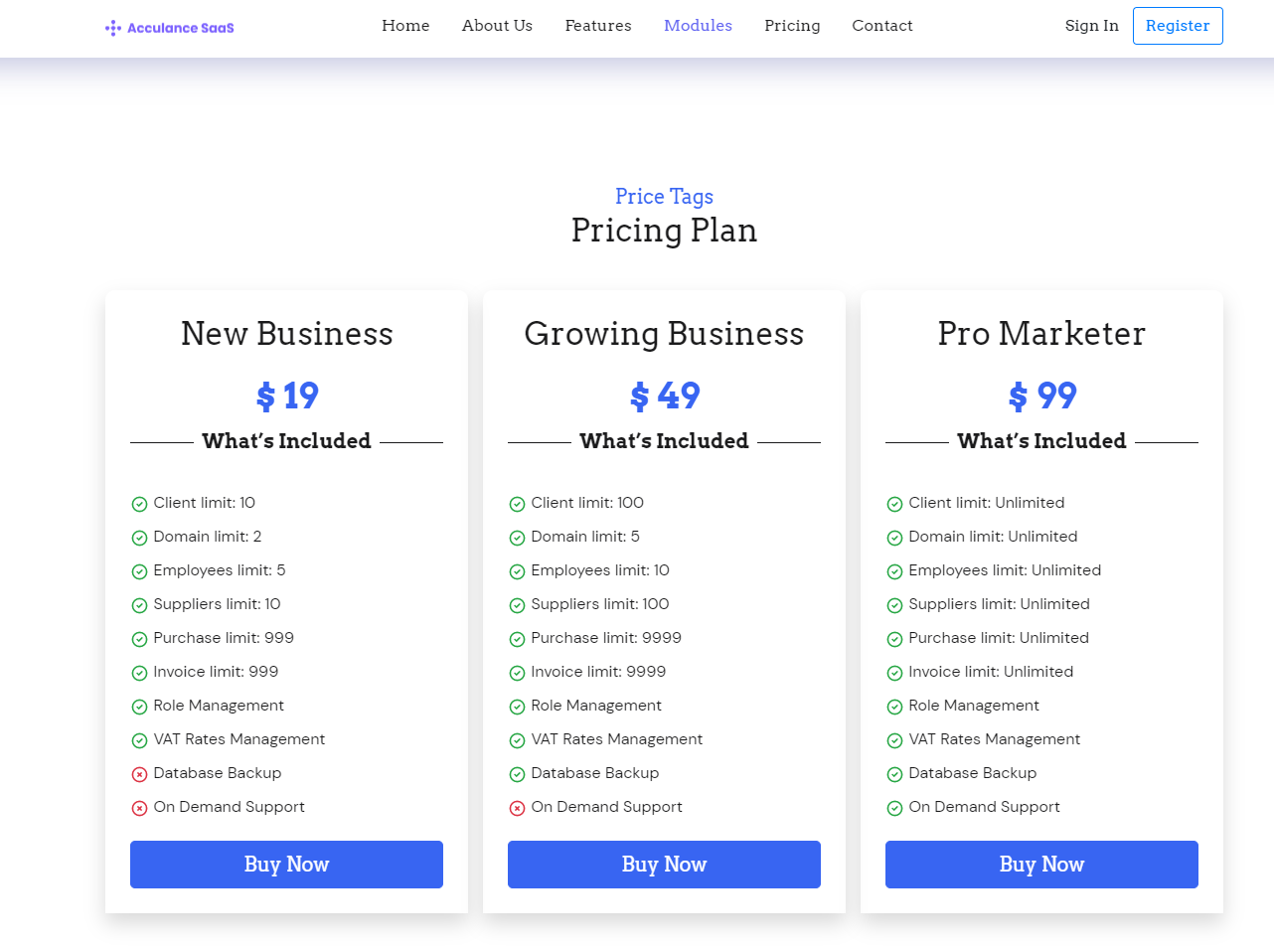Screen capture of a web page displaying the pricing plans for Aculance SAAS, a software-as-a-service platform. 

### Top Navigation Bar:
- **Upper Left**: The logo and name "Aculance SAAS" spelled "A-C-C-U-L-A-N-C-E".
- **Top Center**: Standard navigation buttons: "Home," "About Us," "Features," "Modules," "Pricing," and "Contact."
- **Top Right**: Options to "Sign In" or "Register."

### Main Content Area:
In the center, three vertical, rectangular white blocks present various pricing plans, each detailing the name, price, and included features.

1. **Plan 1: New Business**
   - **Price**: $19 (in blue font)
   - **Included Features**:
     - Client limit
     - Domain limit
     - Employee limit
     - Supplier limit
     - Purchase limit
     - Invoice limit
     - Role management
     - VAT rates management
     - Database backup
     - Online demand support
   - Additional features indicated by green check marks, and some features not included are left unmarked.
   - **Button**: "Buy Now" (in a blue rectangle, white font)

2. **Plan 2: Growing Business**
   - **Price**: $49
   - Structure and feature listing similar to the "New Business" plan, with more features marked by green check marks.

3. **Plan 3: Pro Marketer**
   - **Price**: $99
   - The most comprehensive plan, with all items from the features list marked by green check marks.
   
Each pricing plan block consistently follows the same layout, ensuring clarity and easy comparison for potential customers.